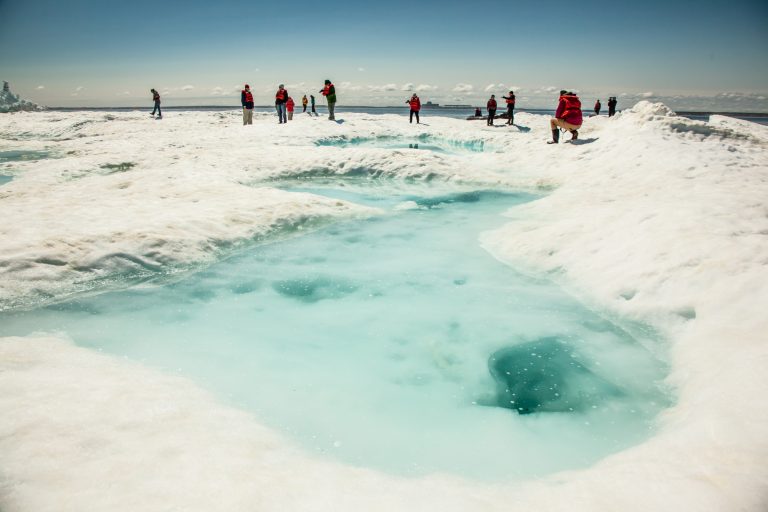This photograph captures a scene in Antarctica featuring a glacial landscape dotted with pools of melted ice. In the foreground, a prominent pool of crystal-clear water reveals a large hole that penetrates deep into the ice, possibly extending down to the ocean below. Surrounding the pool, a group of researchers clad in red and orange safety vests, some with large backpacks, engage in various activities. A few are sitting on portable stools, possibly ice fishing, while others stand and converse, pointing at different features of the icy terrain. The snowy surface stretches toward the horizon, where the white expanse meets a blue sky filled with clouds. In the background, the snowy banks eventually give way to a distant body of water, which is also dotted with research ships, hinting at the researchers' point of origin. The image beautifully contrasts the stark, white snow with the deep blue of the sky and the water, capturing both the isolation and the activity in this frozen environment.